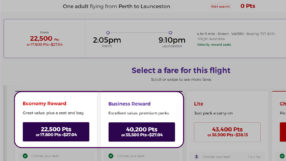The image appears to be a slightly blurry screenshot of a flight booking interface. In the upper right-hand corner, there's a red notification indicating "0 points." Adjacent to it, there is more text, partially obscured, in black and red font. Below this, a section begins with "From 22,500 points" followed by indistinct text, and clearly displays the available flight times: "2:05 PM to 9:10 PM." To the right of the time frames, additional information in grey and green text is present.

Following this, a directive states: "Select a fare for this flight," accompanied by two main highlighted options within rectangles. The left-hand option indicates in red that it costs "22,500 points." The right-hand option, detailed in purple, is labeled "Business Preferred" and priced at "40,200 points." Additionally, there is an unhighlighted option on the far right listed in red, costing "43,400 points." Each option except for the last one includes a green check mark beneath it.